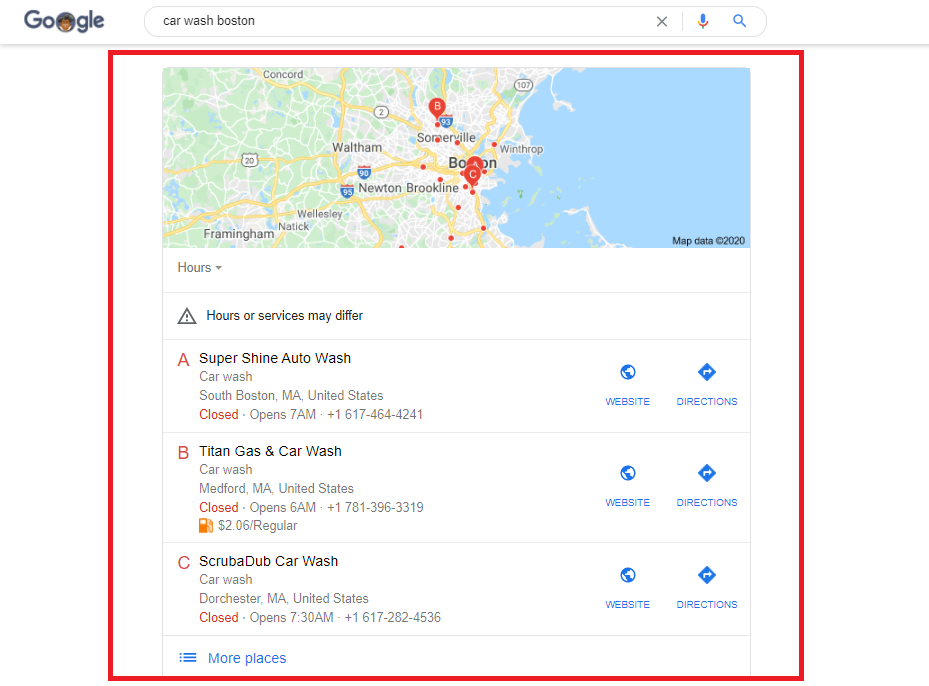A Google Maps inquiry for "Car Wash Boston" reveals a map of the greater Boston area, highlighting three car wash locations with red pins labeled A, B, and C. The map prominently displays the coastline to the east and the surrounding areas of Wellham, Newton, and Brookline to the west of Boston. Below the map, detailed information about each of the highlighted car washes is provided. 

- **A**: Supershine Auto Wash located in South Boston
- **B**: Titan Gas and Car Wash located in Medford, Massachusetts
- **C**: Scrub-A-Dub Car Wash located in Dorchester, Massachusetts

Each car wash listing includes links for both their website and directions. A note specifies that "hours of service may differ," ensuring users are aware of potential variations in operating hours.